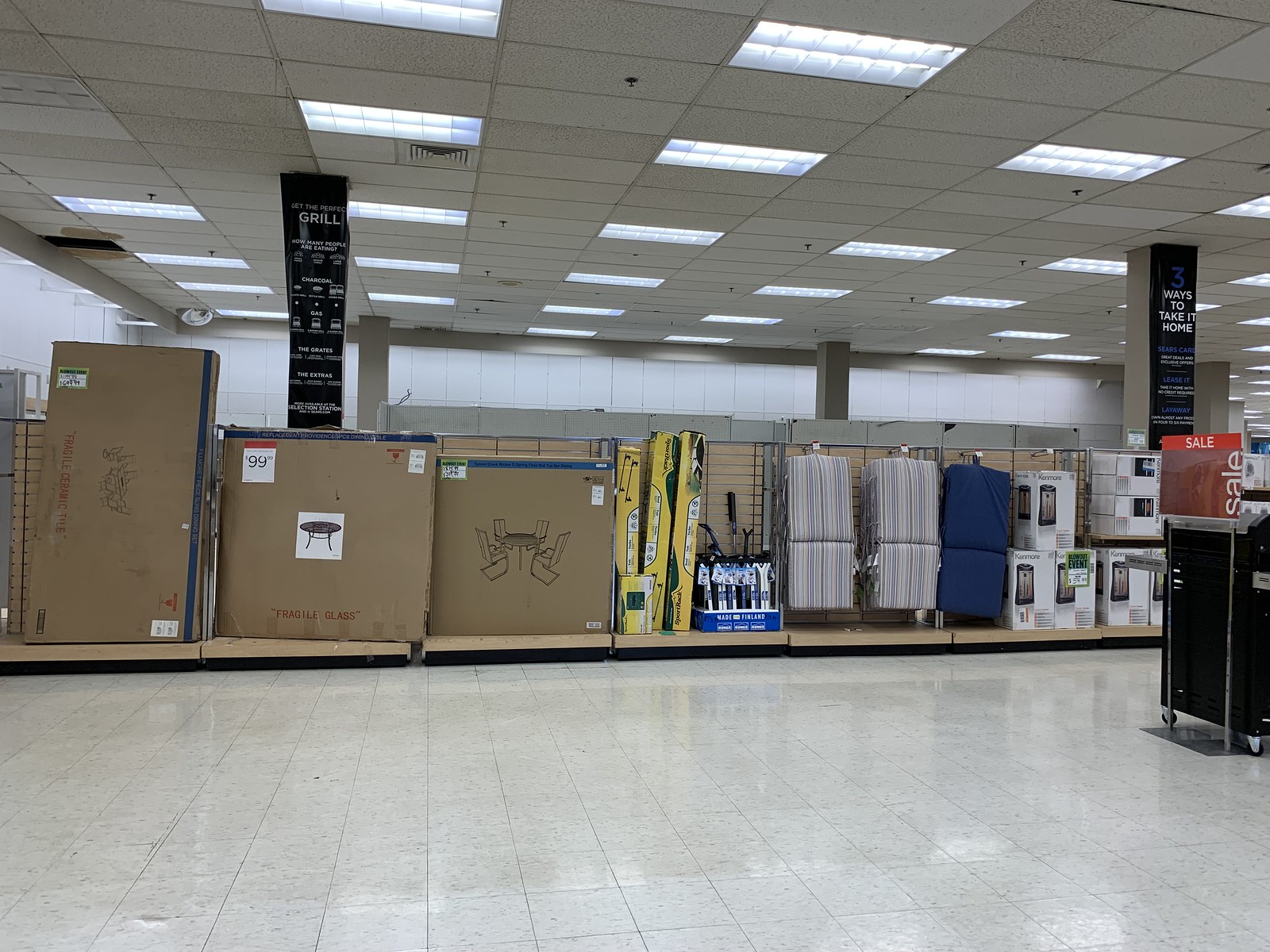This photograph captures the interior of a retail store, likely a Walmart or Target, focusing on the outdoor section. On the right side, there's a prominent red sales sign with white lettering. A large black sign extending from the ceiling to the floor features information about grills, also in white lettering.

In the aisle, various outdoor products are neatly arranged, creating a somewhat sparse but clean appearance. The central display includes tables and chairs, chair cushions, and lanterns. Next to the sales sign on the right is a black metal grill with silver or gray accents.

The store is immaculate, with shiny gray and white tiled floors that enhance the tidy and organized environment.